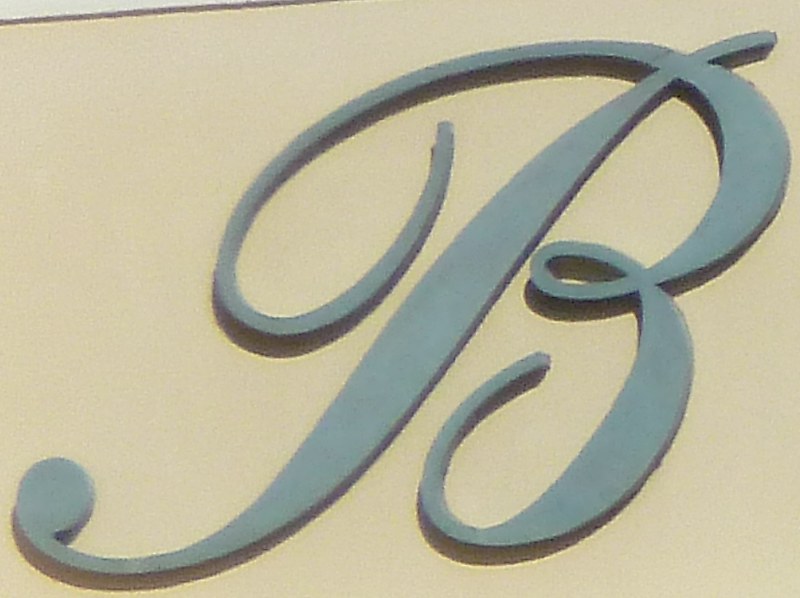This photograph features a beautifully crafted letter 'B' mounted on the exterior of a building. The stylized 'B', rendered in an elegant cursive script, has an almost traditional aura, reminiscent of classic department store signage such as Boscov's. The letter is a pale grayish blue, suggesting it may have experienced some weathering over time, which adds to its vintage charm. The 'B' is notably thick, appearing to be a few inches in depth, which allows it to cast distinct shadows onto the surface of the building. These shadows indicate that the photograph was taken during daylight hours. The backdrop for this striking letter is a building with a darker cream-colored facade, providing a pleasing contrast that makes the 'B' stand out even more. No other letters or signs are visible in this shot, emphasizing the singularity and significance of the letter. The overall condition and style of the 'B' hint at it being an older sign, with the mild fading of its color suggesting many years of exposure to the elements.